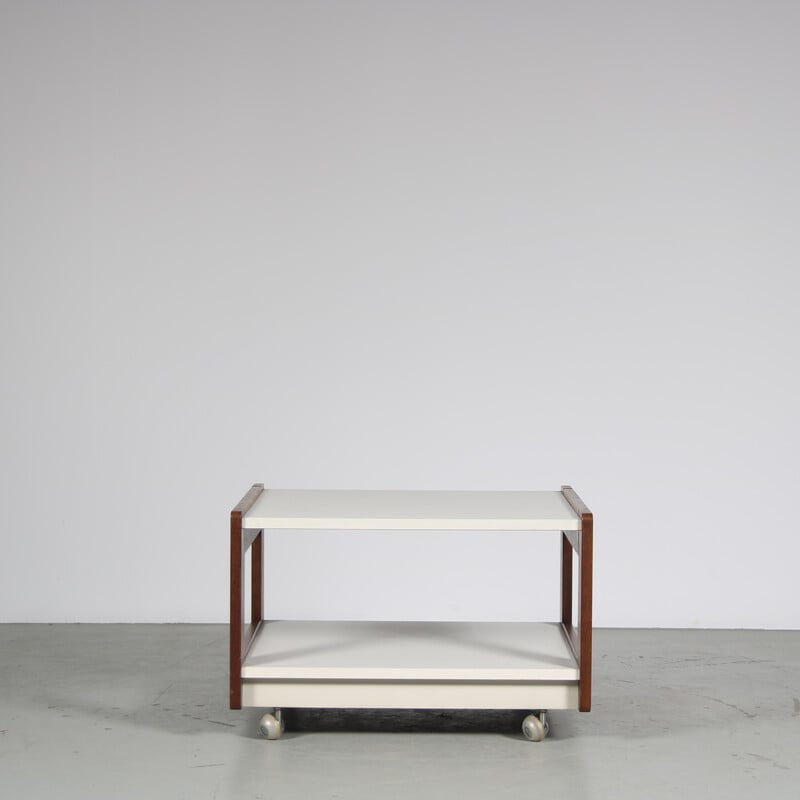This is a detailed photograph of a minimalist rolling cart situated in the middle of an empty room. The cart features a two-layered design with both shelves in a white to creamy white color. These shelves are connected by reddish-brown side frames that might be metal or wood, with square cutouts, and completed by cross posts for additional support. The cart stands on white caster wheels that slightly reflect light, visible against the floor. The room has a hard flooring of a darker gray hue than the walls, adorned with subtle swirls and lines. The background showcases a light gray wall, which appears slightly darker near the top due to shadows. The cart's simplistic and functional design is the focal point, highlighted against the photorealistic, empty grayish environment.